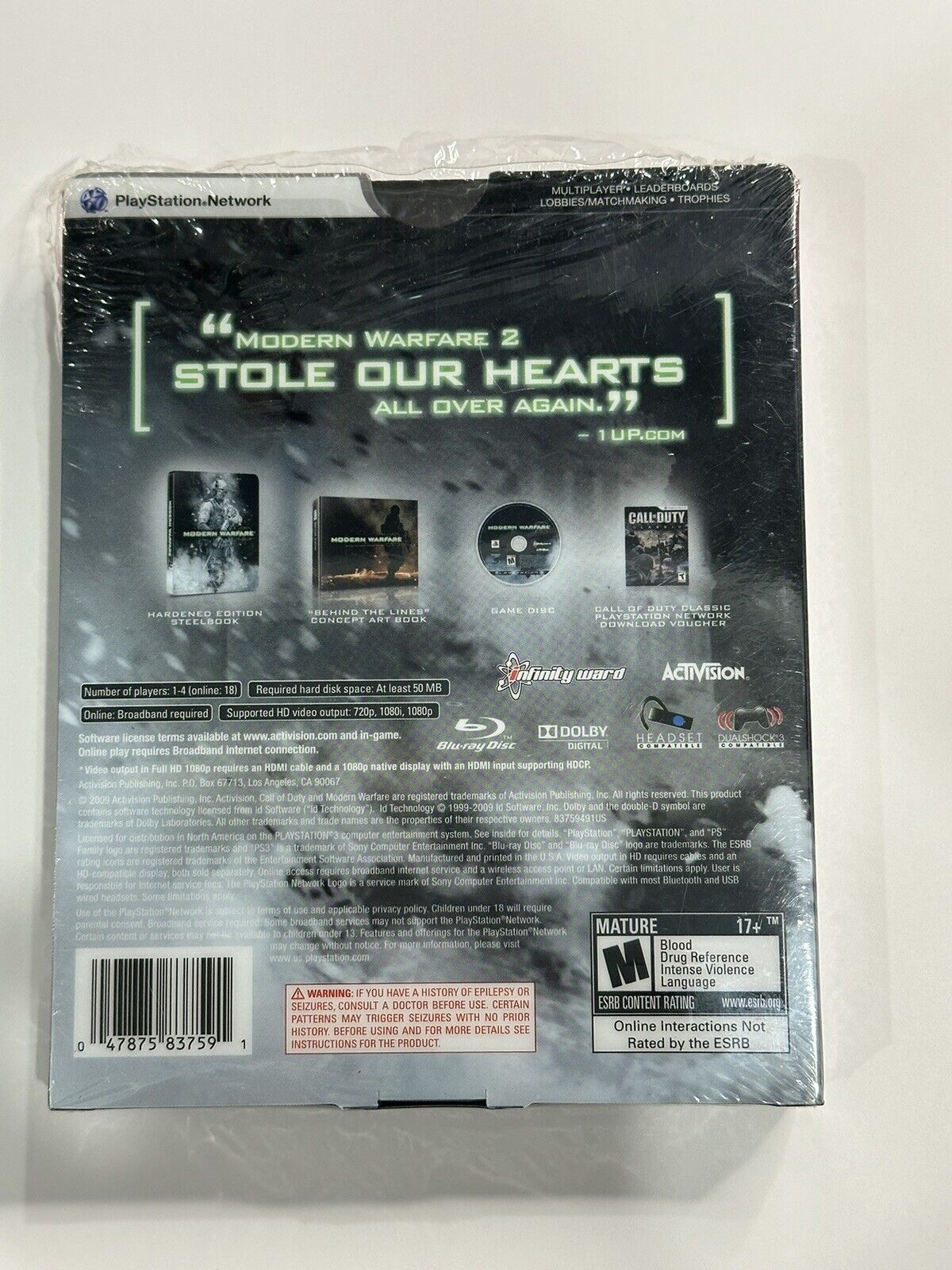This close-up photograph features the shrink-wrapped backside of a PlayStation video game, identified by the PlayStation logo and "PlayStation Network" text in the upper left corner. The game, titled "Modern Warfare 2," includes a quote from 1up.com in light green text that reads, "Modern Warfare 2 stole our hearts all over again." Below the quote, a panoramic view showcases the package contents: a "Hardened Edition" book with a soldier's image and "Modern Warfare" text, a "Behind the Lines" concept art book, the game disc adorned with relevant logos and ratings, and a PlayStation Network Download Voucher for "Call of Duty Classics." The packaging indicates that the game supports resolutions of 720p, 1080i, and 1080p, and is designed for 1-4 players offline or up to 18 online, requiring 50 MB of disc space. The mature rating (M) for the game, due to blood, drug references, intense violence, and language, is prominently displayed, alongside a barcode and a mostly black and smoky gray design. The entirely wrapped game appears to be placed on a white background, likely on a table, ready for purchase.